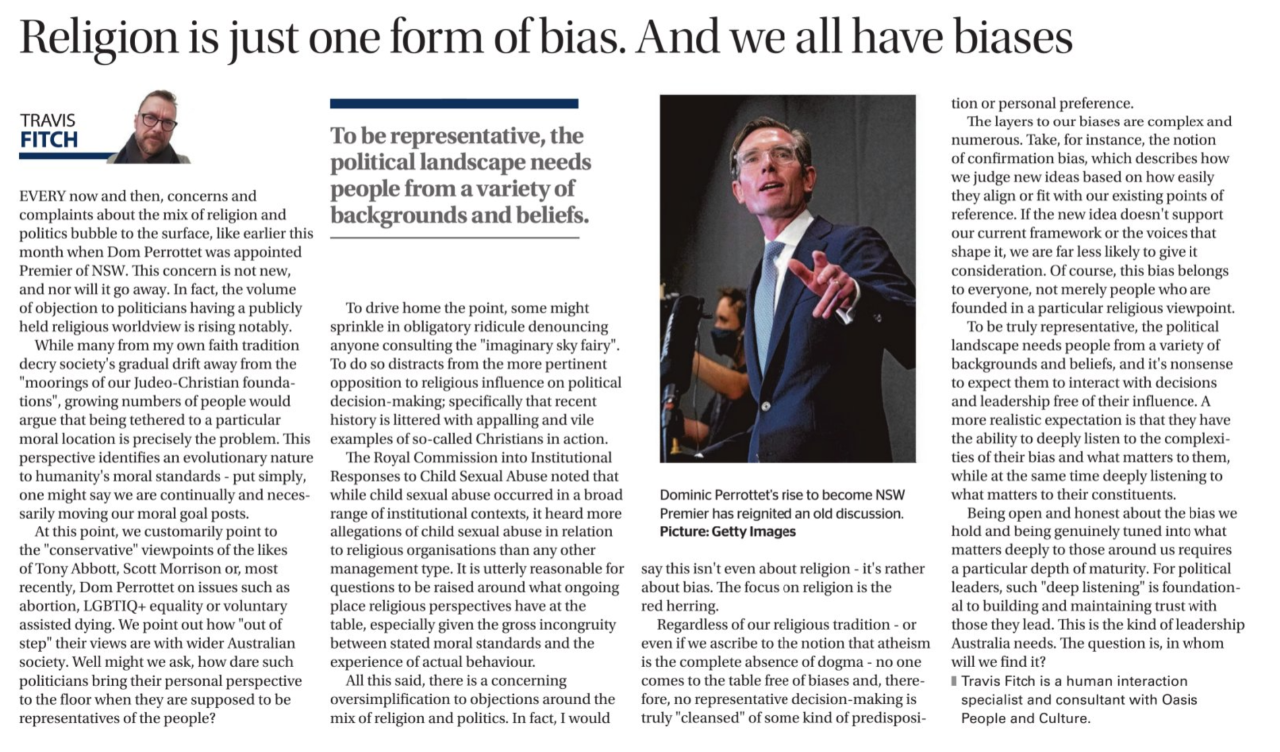The image features a newspaper article prominently titled "Religion Is Just One Form of Bias." The header emphasizes the universality of biases among individuals. Below the headline, on the left-hand side, is the name "Travis Finch," written in bold, all-caps text with a thick underline.

Next to the name is a photograph of a white male with short, slightly spiky hair and a goatee, his head tilted to the side. He is wearing a scarf around his neck.

To the right of this photograph is a section of the article in large print. It reads: "Today, to be representative, the political landscape needs people from a variety of backgrounds and beliefs." This section is separated by a line and a notable amount of space from the rest of the text. Above this segment is a thick line running the width of the column.

Further to the right is another photograph of a man in a business suit, appearing to be in his 40s, possibly wearing glasses, a tie, and seemingly pointing towards something in the image. This individual also appears to be a white male.

The article itself is divided into four columns, each filled with paragraphs elaborating on the theme introduced by the headline.